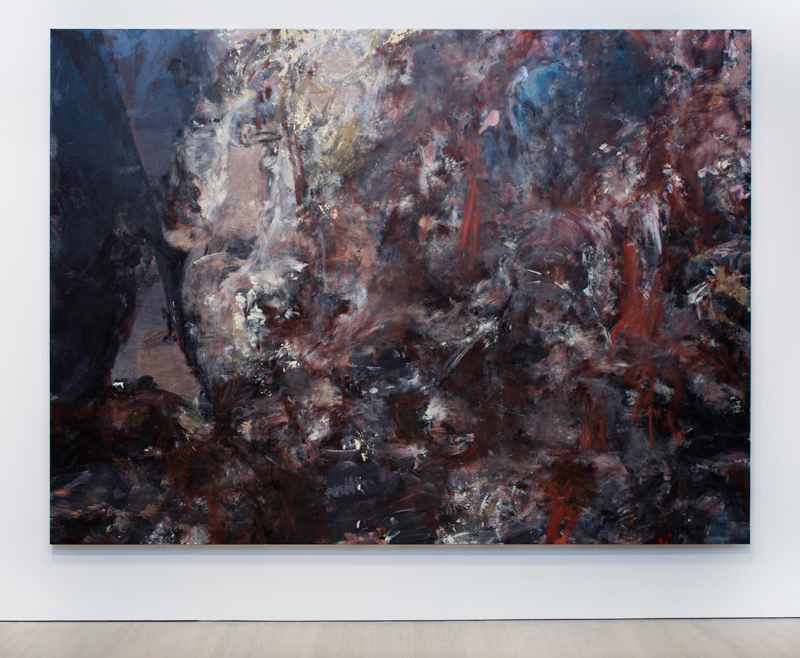This photograph captures a large, extremely abstract painting that hangs in a gallery or museum. The painting is characterized by chaotic brush strokes that seem to emanate in all directions, giving it a tumultuous and dynamic feel. The colors are predominantly dark, with various shades of blue, black, and gray saturating the edges and corners, evoking a sense of ruin and decay. The bottom right corner is particularly dark and foreboding, featuring deep reds and blacks. As one's eye moves towards the center and upper portions, lighter hues begin to emerge—whites, yellows, and creams battle for space amid the chaos, with hints of peach on the left side. This gradation forms an implied diagonal division, suggesting a hill stretching from the bottom left to the top right. Overall, the painting conveys a post-apocalyptic aura with its dingy, dirty palette and intense, disorderly strokes, leaving form and meaning entirely up to the beholder's interpretation.